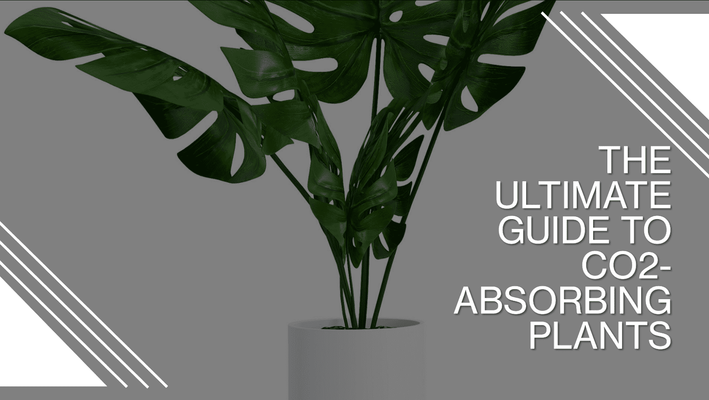The image is a horizontally oriented digital graphic, potentially a PowerPoint title slide, featuring a detailed depiction of a potted plant in the center. The plant, standing at an estimated height of three to five feet, has numerous green leaves characterized by small holes and long, gated stems. The plant is housed in a cylindrical gray vase that blends seamlessly with the predominantly gray background, which is accented by a geometric design of white stripes and triangles, particularly noticeable in the bottom left and top right corners. The text on the right-hand side of the image, in large, capitalized white font, reads "The Ultimate Guide to CO2 Absorbing Plants," effectively capturing the essence of the graphic's purpose. This highly stylized and potentially digitally rendered or edited image, with its smooth, polished appearance, suggests it is part of a professional graphic design project or stock image collection for presentations.